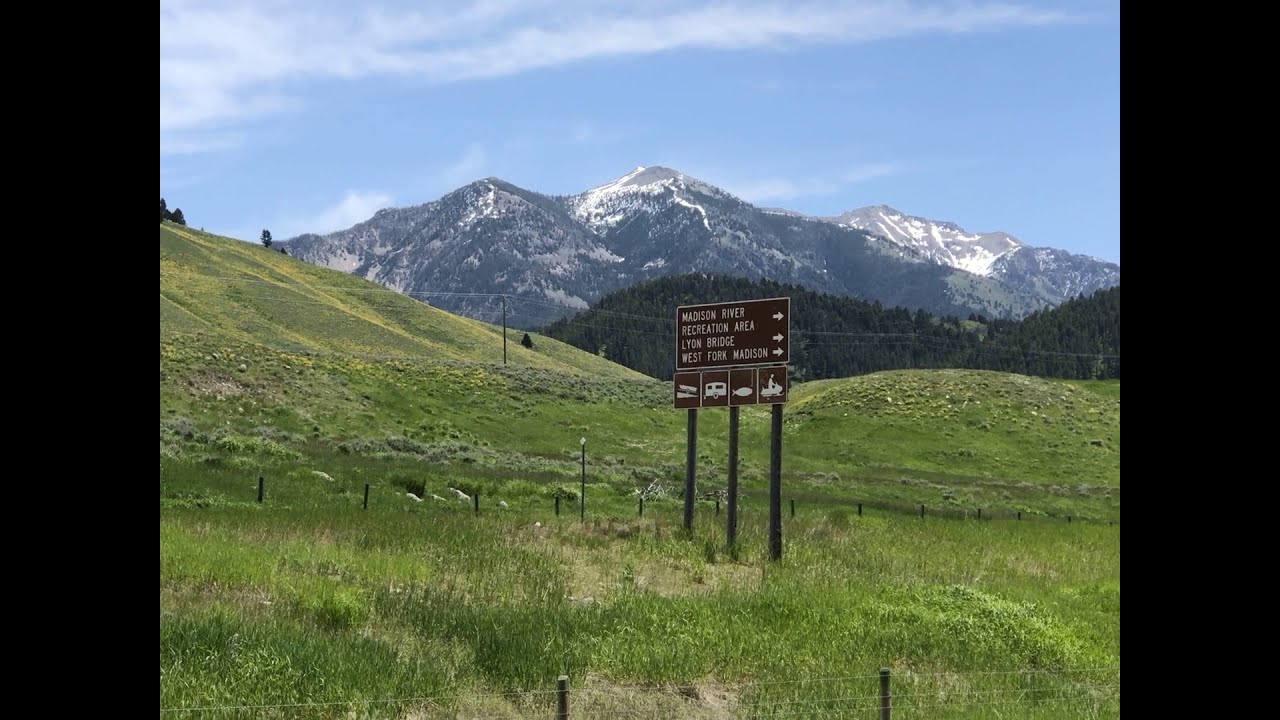This is a wide, rectangular photograph capturing a picturesque rural, mountainous valley, likely near the Rocky Mountains. Dominating the foreground is a green, grassy field interspersed with gray patches and long, soft shoots. A barbed wire-style fence with gray poles and white wires runs along the bottom of the image. 

Central to the scene is a brown directional sign, mounted on three metal poles, displaying "Madison River Recreation Area," "Lion Bridge," and "West Fork Madison." It also features icons for jet skiing, fishing, and camping. Behind the sign, undulating grassy hills give way to a distant range of snowy-topped mountains with dense greenery in the middle featuring trees with green foliage, possibly pines.

Throughout the landscape, power lines and telephone poles are visible, adding a touch of rural infrastructure to the natural setting. The sky above is a light blue, adorned with gentle, misty white clouds, suggesting the photograph was taken during the daytime. The thick black rectangles on the left and right edges of the image suggest it has been cropped. This tranquil scene is a beautiful blend of natural and man-made elements set against a stunning mountainous backdrop.